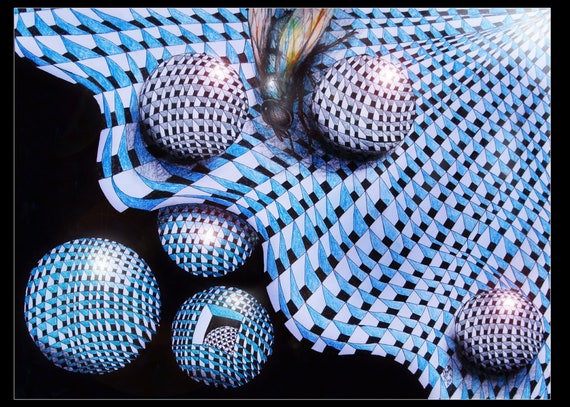The image is an abstract, slightly rectangular, and horizontal color pencil drawing set against a closely bordered black backdrop. The artwork features six 3D spheres adorned with a plaid-like pattern of dark blue, light blue, and black. These spheres appear on a curvy planar surface that flows diagonally from the top right corner to the bottom left, creating a dynamic visual effect. This surface, covered in a similar geometric pattern, sometimes obscures parts of the spheres, with one sphere partially hidden underneath. A housefly with a black face and blue body, sporting clear white, green, and red wings, is depicted on one of the spheres near the top center. The image is illuminated by rendered light, accentuating the shiny texture of the spheres. A bright white light in the very right corner contrasts with the dominant blue hues, contributing to the artwork's ethereal ambiance.